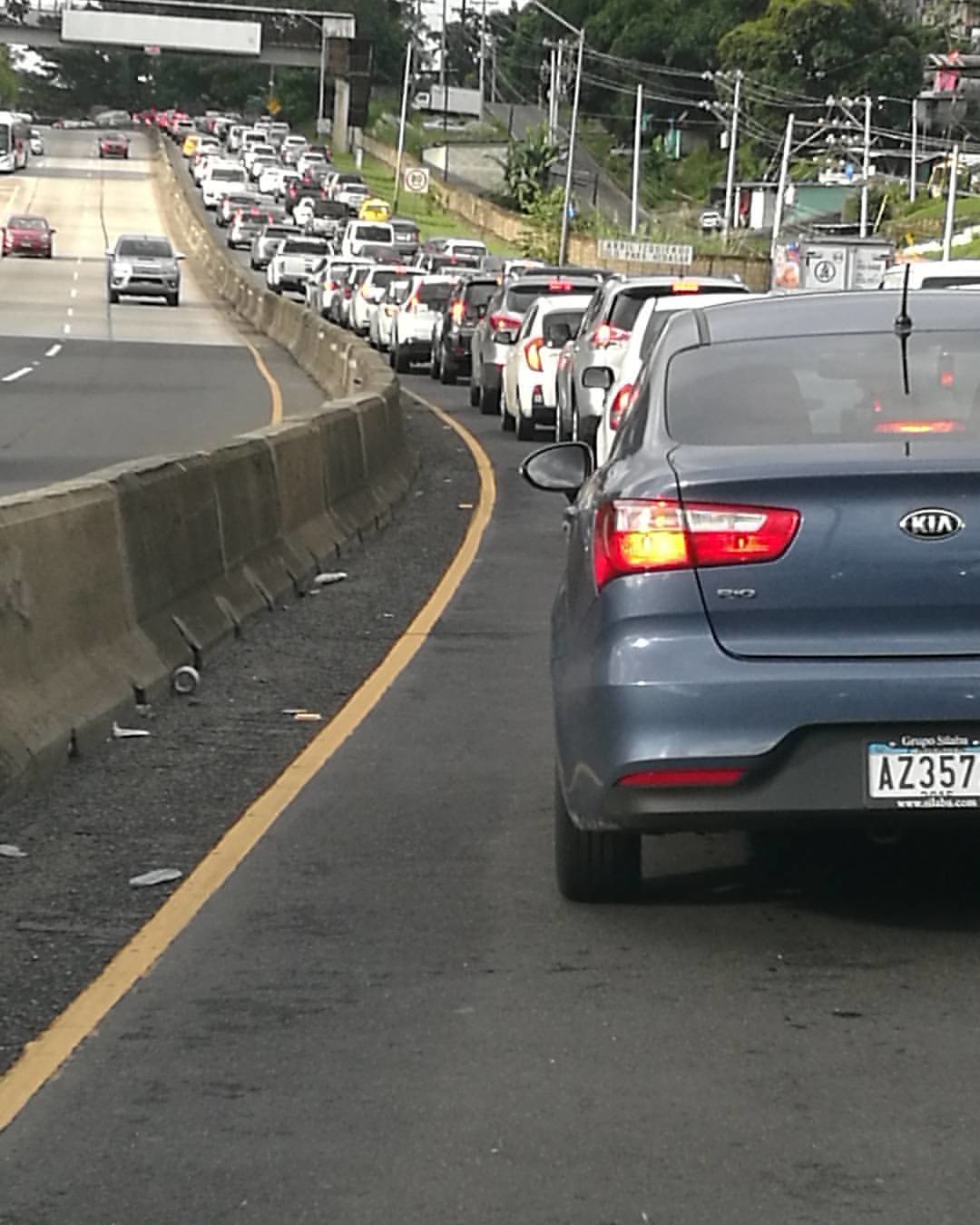View from the driver's seat captures the frustration of a bumper-to-bumper traffic jam on a three-lane highway. The camera is positioned in the left-most lane of the congested side, highlighting the stark contrast with the opposite lanes on the left which flow freely with just three cars visible. A small hill looms ahead, adding to the sense of slow, arduous progress. On the right-hand side, power lines stretch overhead, bordering a mix of trees and residential buildings, hinting at the proximity to a neighborhood. The overall scene encapsulates the frustrating halt of a routine commute.